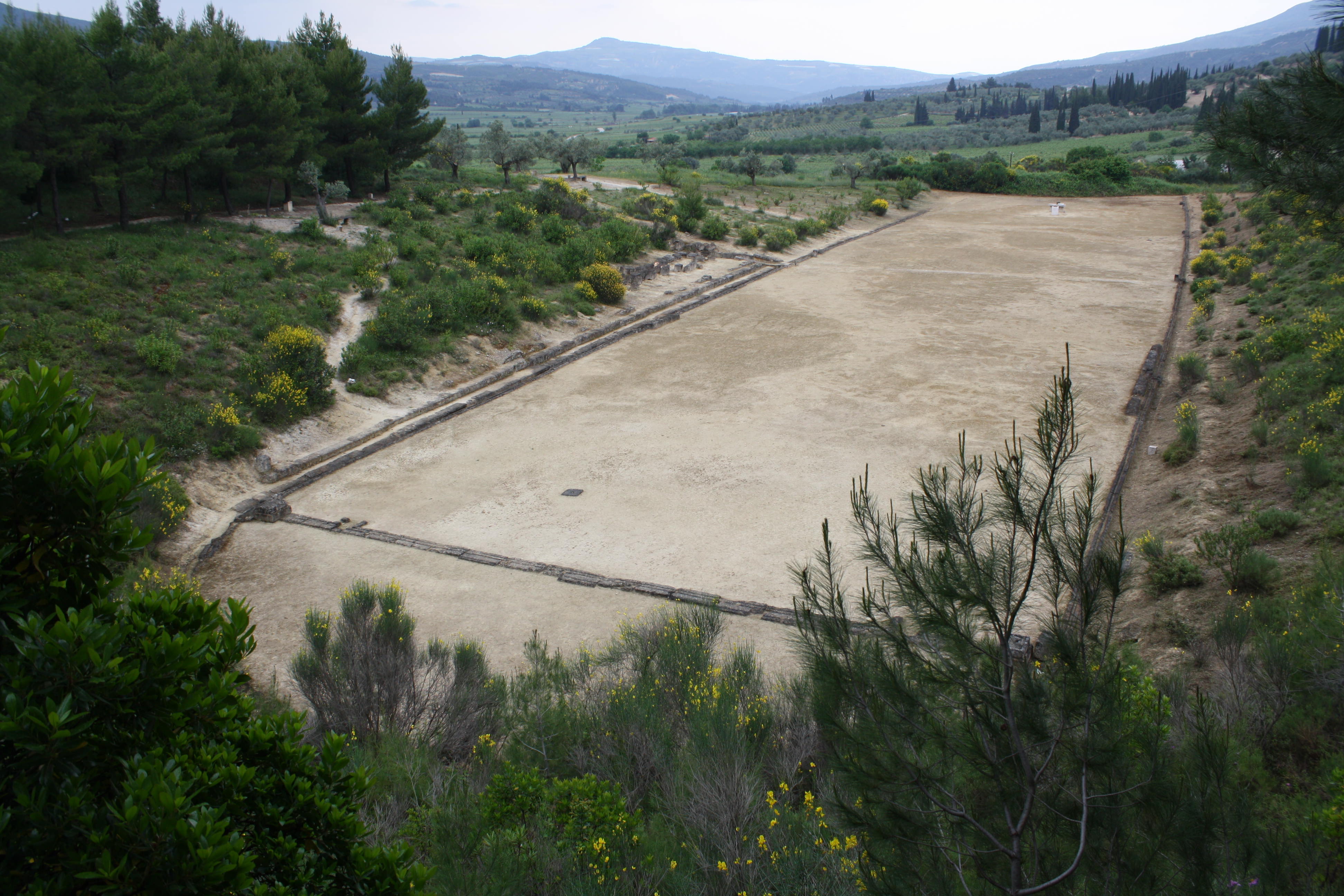This detailed photograph, captured from an elevated vantage point, offers an aerial view of a rectangular plot of land amidst a predominantly forested area. The setting is outdoors during the daytime, with the photographer positioned perhaps on a hill. Central to the image is a distinctly rectangular, bare plot of soil, appearing to be prepared for some future use, resembling a stadium or sports field. The soil patch, mostly off-white with brown splotches, is smooth and clear of any vegetation.

Surrounding this cleared land are gentle slopes adorned with flowers, wildflowers, and weeds. The slopes give way to dense clusters of evergreen trees, which frame the plot on all sides: prominently in the foreground, top left, and bottom right corners of the image. Further beyond, the landscape transitions into hills and valleys covered with more trees and grass.

In the distance, majestic blue mountains rise against a backdrop of a sky painted with gradients of white and blue; the sky appears white over the central part of the image and transitions to a deeper blue towards the edges. This pristine setting captures the beauty of nature and the mystery of the cleared, rectangular land at its heart.